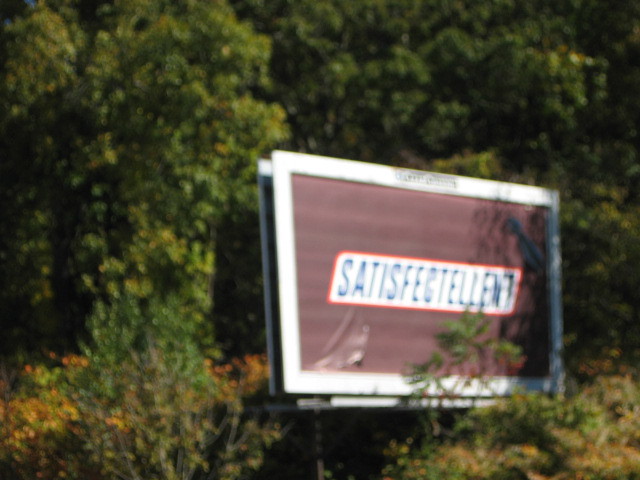This blurry outdoor photograph captures a large white-framed billboard surrounded by a dense cluster of trees. The trees, dominating the entire frame, exhibit a range of green hues, with some leaves transitioning to yellow, orange, and red. The billboard, positioned in a three-quarter profile facing slightly to the right, prominently features an advertisement with a dark chocolate brown background. At its center is a slightly angled white rectangle, bordered by a thin red outline and blue text that reads "Satisfectalent" (S-A-T-I-S-F-E-C-T-E-L-L-E-N-T), echoing the font and style of Snickers candy bars. Notably, there's a small rip at the lower left corner of the billboard, and some tree branches partially obscure its view.